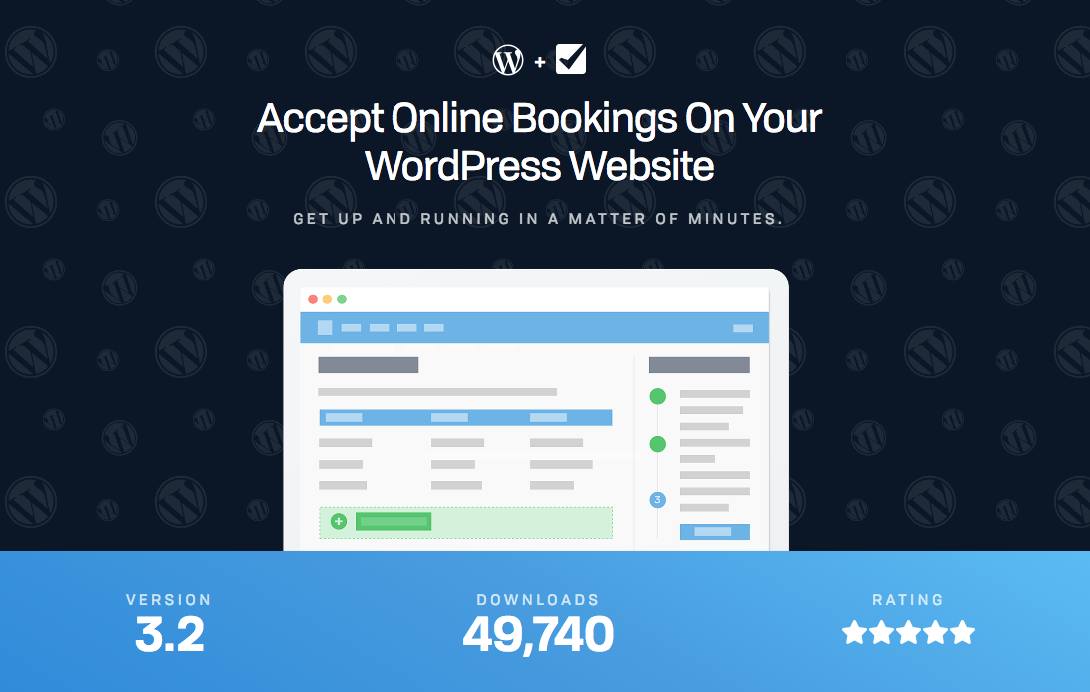This digitally created screenshot features a predominantly black background, adorned with numerous floating gray circles, each with a black "W" at its center, which suggests these could be representative of WordPress logos. Prominently positioned at the top of the image is a call to action: "Accept online bookings on your WordPress website. Get up and running in a matter of minutes."

An illustrated computer screen is displayed below the text, reinforcing the digital nature of the topic. At the bottom, there is a blue border containing key information in white typography: "Version 3.2," "Downloads 49,740," and a perfect "5 out of 5 stars" rating.

The image has a landscape orientation, wider than it is tall, and lacks any photographic elements, depicting neither people, animals, plants, nor vehicles. Its clean, uniform design focuses entirely on conveying information about a WordPress booking plugin in a visually cohesive manner.